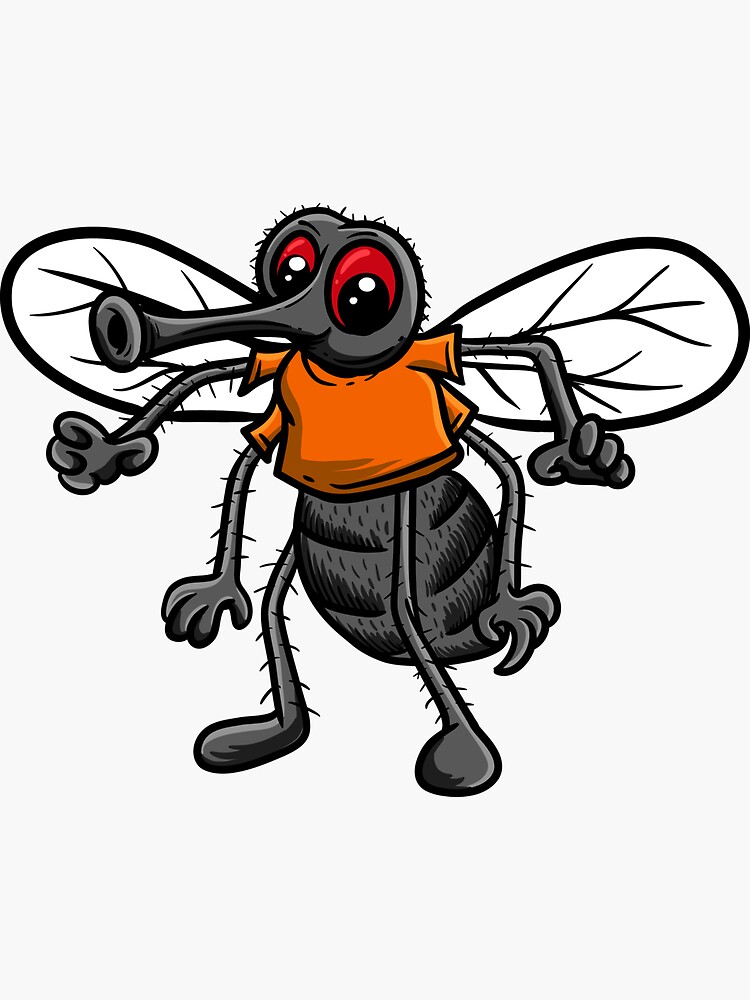The image is a highly detailed, close-up, colored illustration of a cartoon insect resembling a fly. The fly is depicted with a dark gray and black body, featuring prominent red, bulging eyes that look upwards. It has a distinctive tubular nose pointing to the left of the image, and it wears an orange shirt, fitted with multiple short sleeves accommodating its four arms and two legs. The fly appears to be standing on two round feet, with its elliptical-shaped abdomen hanging below the shirt. The fly has narrow elliptical wings, outlined in black with internal black veins, giving a clear yet slightly transparent appearance. The background of the image is completely white, emphasizing the clarity and brightness of the scene without any additional characters, text, or artist signature. The overall image is crisp, vividly colored, and well-lit, showcasing the fly's detailed and expressive design.